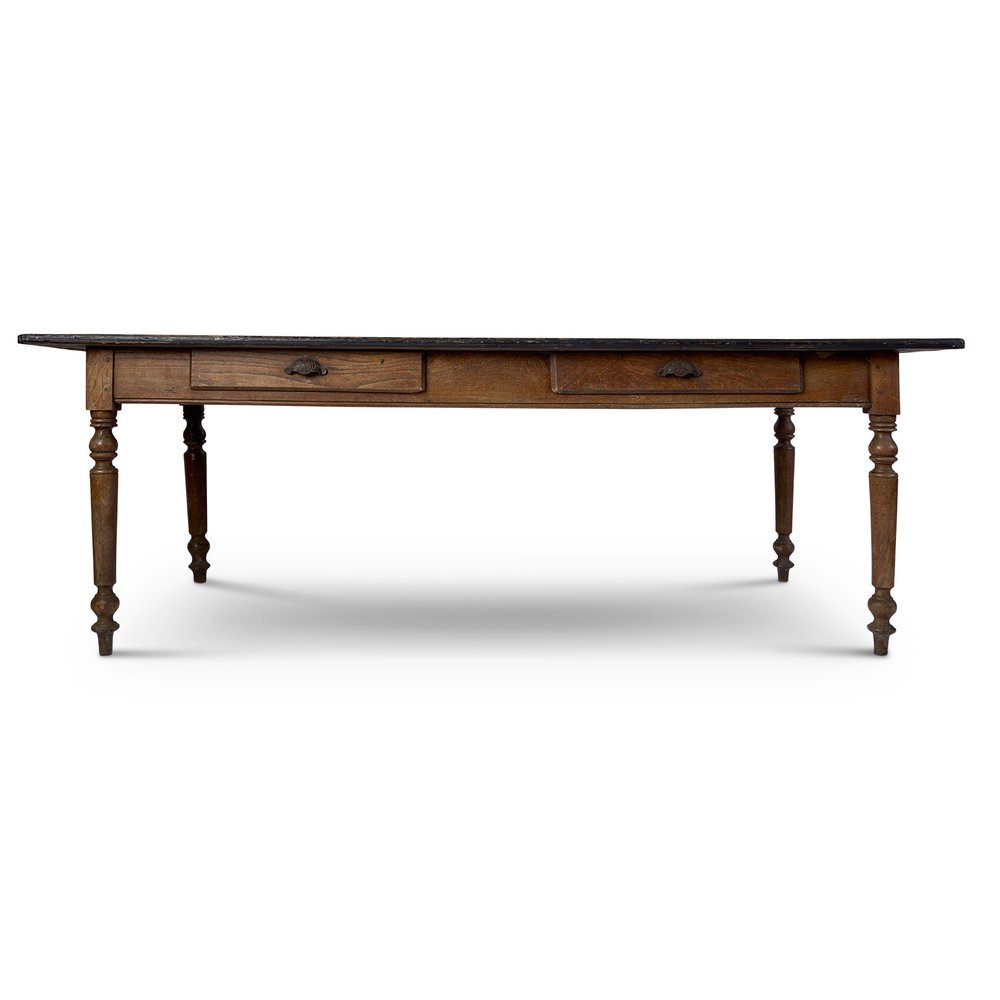The image is a product photo of a wooden coffee table set against a minimalist white background, emphasizing its design. The table features a dark brown top that contrasts with the medium-toned wooden body. The side view reveals two narrow drawers with bronze handles, located just below the tabletop. The table stands on four decorative legs, each shaped with a mix of cylindrical and rounded elements, creating a curvy, ornate appearance. A small shadow is visible under the table, adding depth to the otherwise stark white void surrounding it.